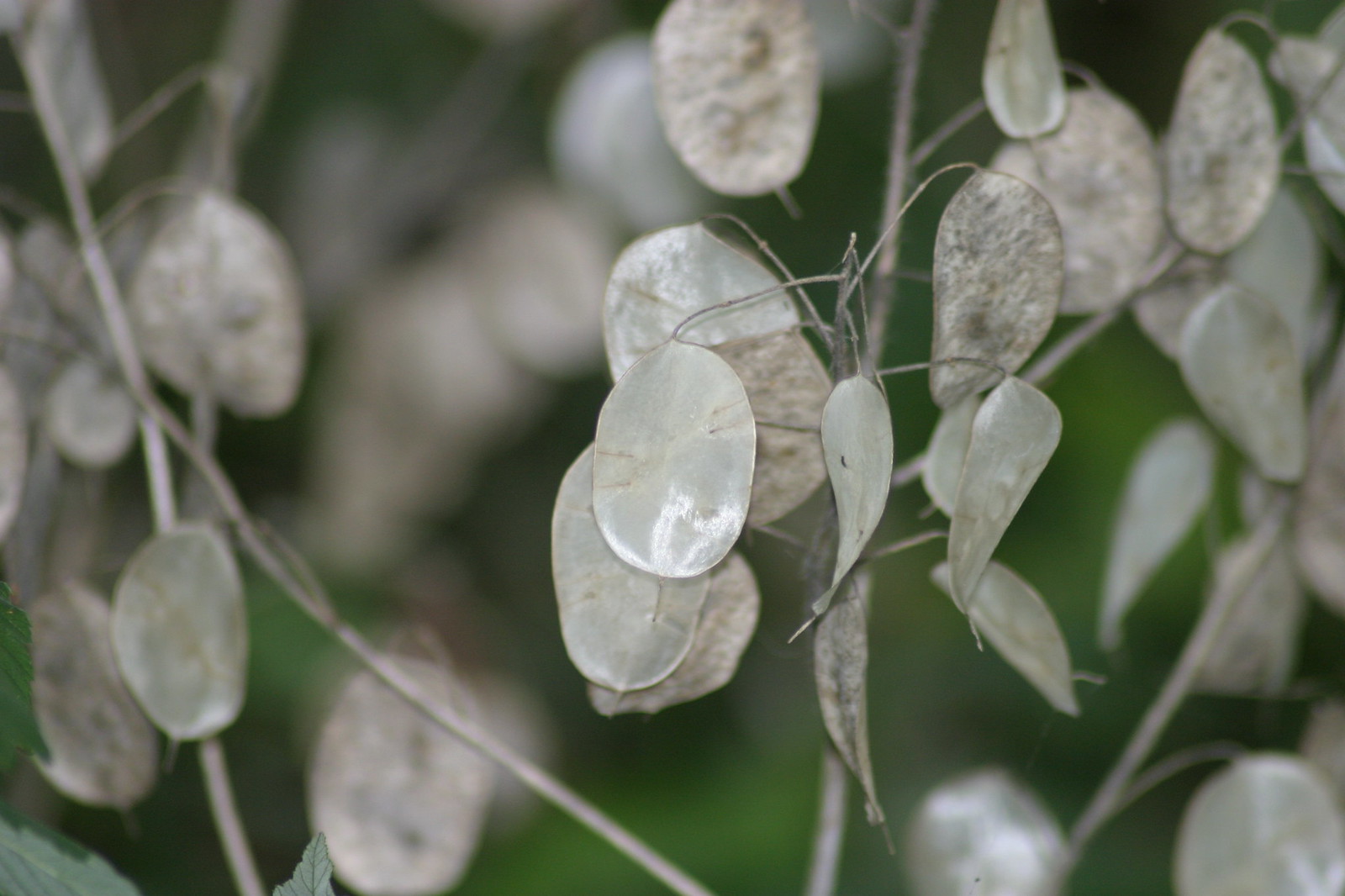The photograph is a rectangular image capturing a natural outdoor scene, likely within a garden. The background is blurred green vegetation, which creates a subtle, out-of-focus backdrop that accentuates the central subject. The focus of the photograph is a distinctive plant known colloquially as a money plant. The leaves of the plant are disc-shaped and possess a unique pearly white color, almost translucent with a grayish hue, appearing light and shiny like pearls. These leaves dominate the image, their delicate texture standing out among some scattered branches and stems that extend across the center of the frame. Additionally, within this plant, there's an intriguing element that might be a spindly-legged insect, possibly a grasshopper, blending so seamlessly it could almost be mistaken for one of the white leaves. The overall color palette of the photograph includes various shades of green, from the light green and greyish leaves to the subdued green and brown of the background foliage, hinting at an autumn setting. The scene is bathed in natural daylight, capturing the quiet elegance of this garden space.